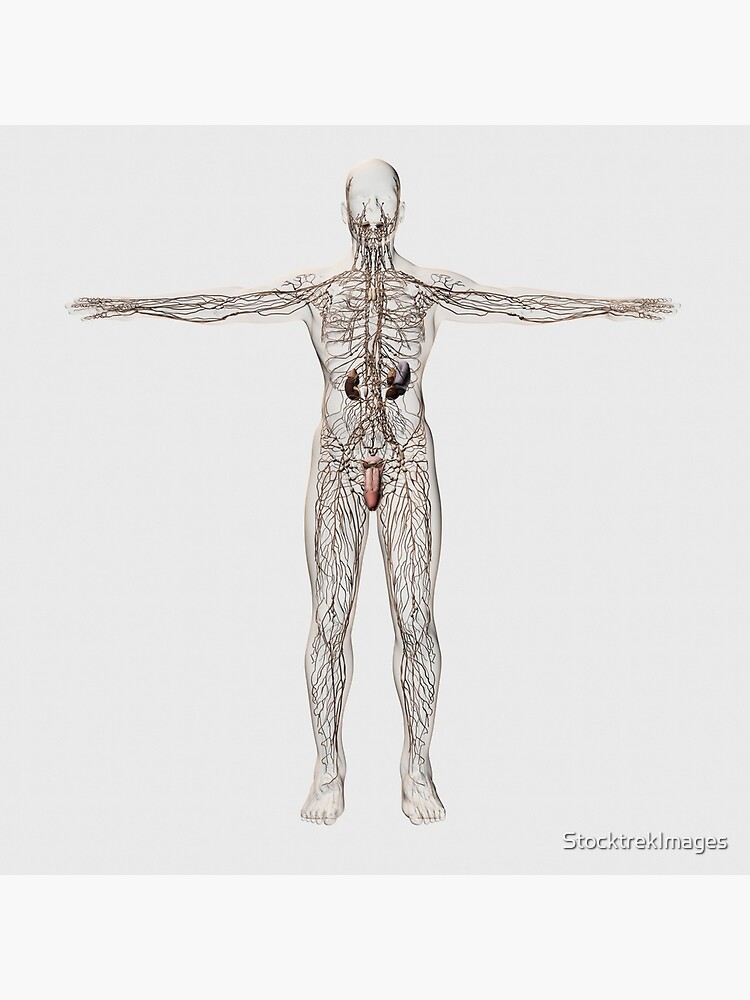This image is a detailed, pencil-like illustration of the human male body, possibly extracted from a medical textbook or an online source. The figure stands upright with legs slightly apart and arms stretched horizontally, resembling a standard anatomical pose. The drawing is set against a gray square background with the label "Stock Trek Images" imprinted in white at the bottom right. The depiction is predominantly of the circulatory system, with intricate lines representing arteries, veins, and nerves spanning throughout the transparent outline of the body from the head to the toes and fingertips. Notable anatomical features include visible ribs, although they could also be the vascular patterns around the ribcage, and distinctive details of the external genitalia, which are illustrated in pink for contrast. Internal organs are minimally depicted, showing only the kidneys or possibly another organ within the torso. The face lacks detailed features, apart from an outline suggesting a wide nose. This intricate yet simple representation effectively highlights the vascular anatomy of the human body.